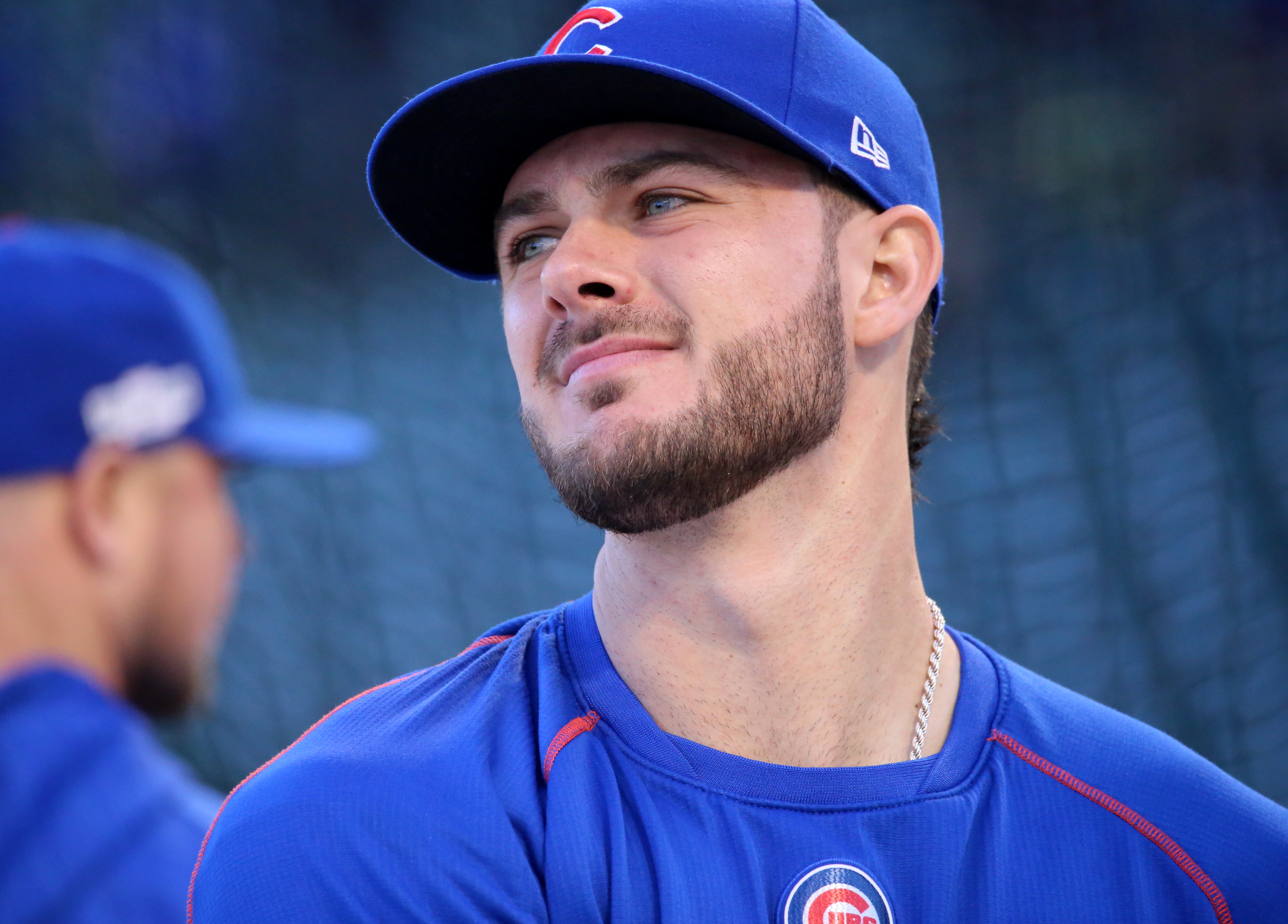The photograph captures two baseball players, both members of the Cubs team, defined by their blue jerseys adorned with red stripes along the shoulders and a prominent white circle logo with a blue border and red "Cubs" lettering on the chest. The central figure, who is in sharp focus, dons a blue baseball cap featuring a large red "C" bordered in white, and a silver chain necklace around his neck. He is a Caucasian male in his 20s or 30s with blue eyes, black hair, and facial hair including a scruffy beard, Fu Manchu, and small mustache. He is gazing off to the left, where the off-screen action seems to attract his attention. Partially visible and out of focus on the left side is another player, similarly attired, but obscured and looking in the opposite direction. The background includes a blue curtain, suggesting the setting might be a dugout or indoor practice area.